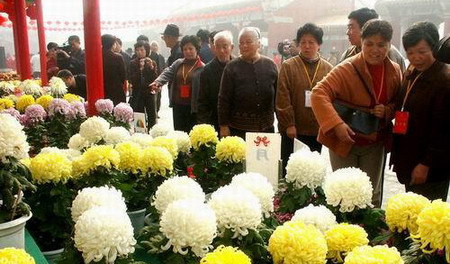The photograph depicts an outdoor scene, likely set in an Asian country, featuring a bustling area where approximately 15 people are gathered. These individuals, appearing to be of Asian descent and mostly older, are lined up and intently observing a vibrant display of flowers. The flowers, which include large-bulbed yellow, off-white, and light pink varieties that look like marigolds or mums, are arranged in numerous pots. The people, dressed in coats suggesting cool weather, are part of an outdoor market or flower sale. Adding to the scene, there are red pillars adorned with ornaments, likely supporting an awning, and in the background, several buildings can be seen, enhancing the context of the lively market environment.